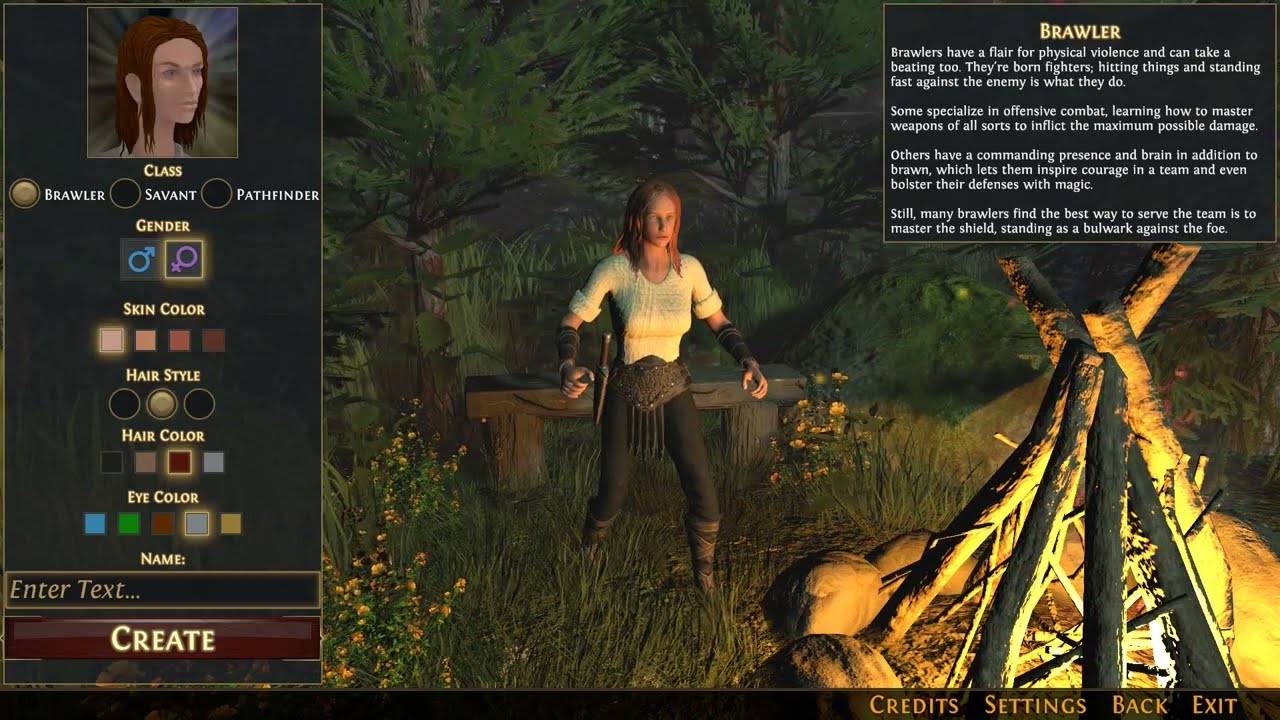This image is a detailed screenshot from a video game displayed on a computer or TV monitor, showcasing a character customization screen set against the backdrop of a vibrant forest scene. In the center, a woman stands by a large campfire, ready for battle. She has brown hair, possibly wet, and is outfitted in a white shirt, tight black pants, a large black belt, black boots, and black gloves. She holds a knife or hatchet, embodying the fierce independence and readiness of a brawler.

On the upper right side of the screen, a black square displays the class information in yellow text that reads "Brawler," followed by detailed white text explaining the characteristics of the class. The text describes brawlers as having a flair for physical violence, resilience, and varied abilities such as offensive combat, inspiring teammates, and defensive tactics involving shields.

To the left, a vertical black strip features the customization menu. At the top is a head profile of the character class with the word "Class" underneath, followed by the options to choose between "Brawler," "Savant," and "Pathfinder." Below these options, users can select the gender, skin color, hairstyle, hair color, eye color, and name for their character. Currently, the brawler class is selected, with a female character of pale skin and burgundy hair. The control options to further personalize the character are clearly outlined.

The tranquil forest setting in the background includes green grass, trees, bushes, and a gray stone bench, suggesting an evening time ambiance. The lower right side of the screen also includes credit and exit controls, adding to the immersive customization experience.